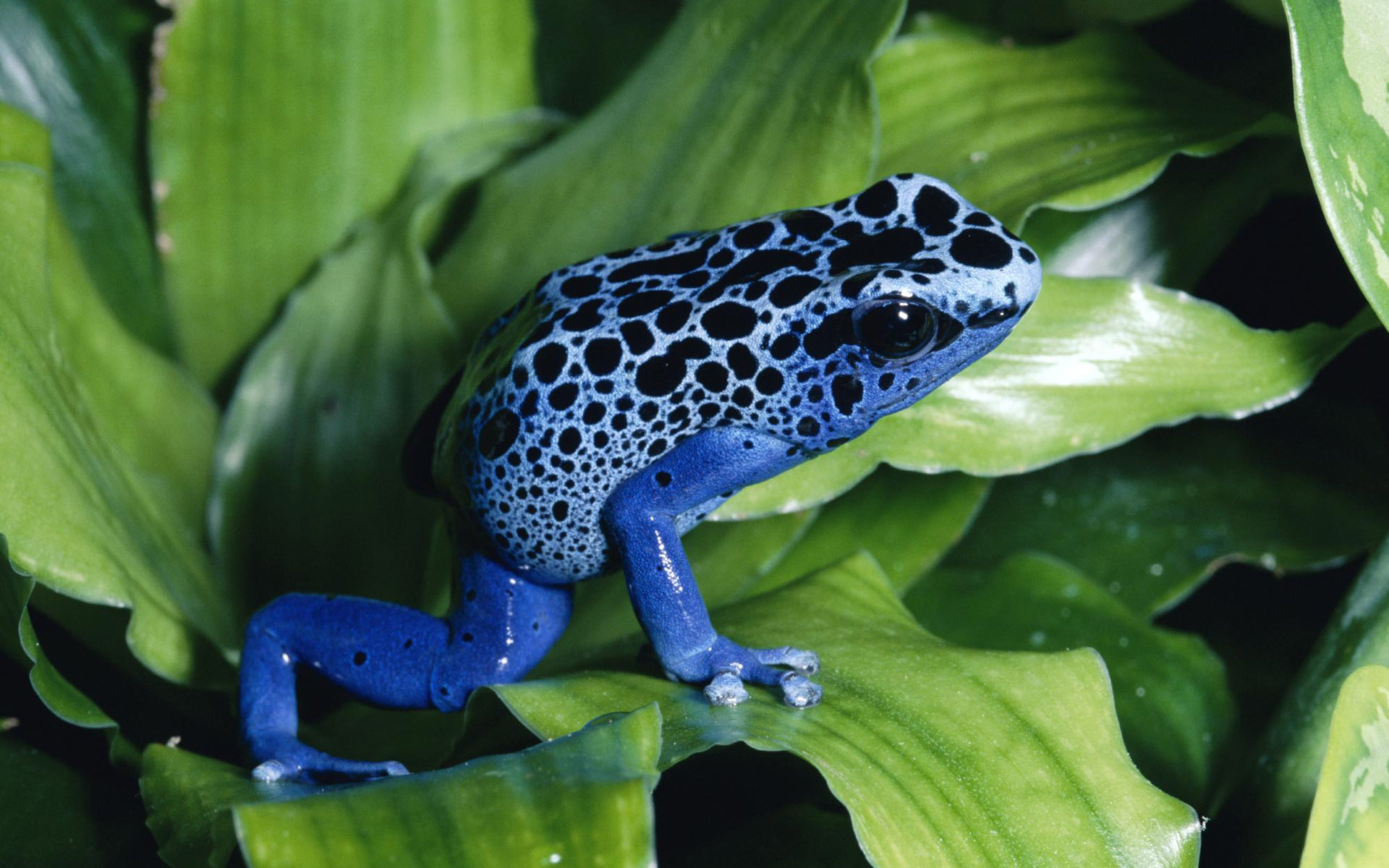The photograph captures an intensely blue, spotted frog poised on a vivid green plant amidst a lush, rain-kissed rainforest backdrop. The frog is centrally positioned, offering a right-side profile view that prominently displays its strikingly large, black eye with a white reflection. Its vibrant blue legs feature a few small black spots, while the lighter blue of its body is adorned with an array of larger, varied black spots, some circular and some elongated, heavily concentrated along the top of its head and back. The plant it rests on has smooth, waxy, spear-shaped leaves with distinct vertical ridges, radiating from a central point. The background reveals more of these leaves, dripping wet and slightly blurred, enhancing the rainforest ambience. The overall scene exudes the freshness of a recent rain, intensifying the intricate details and vivid colors of the frog and foliage.